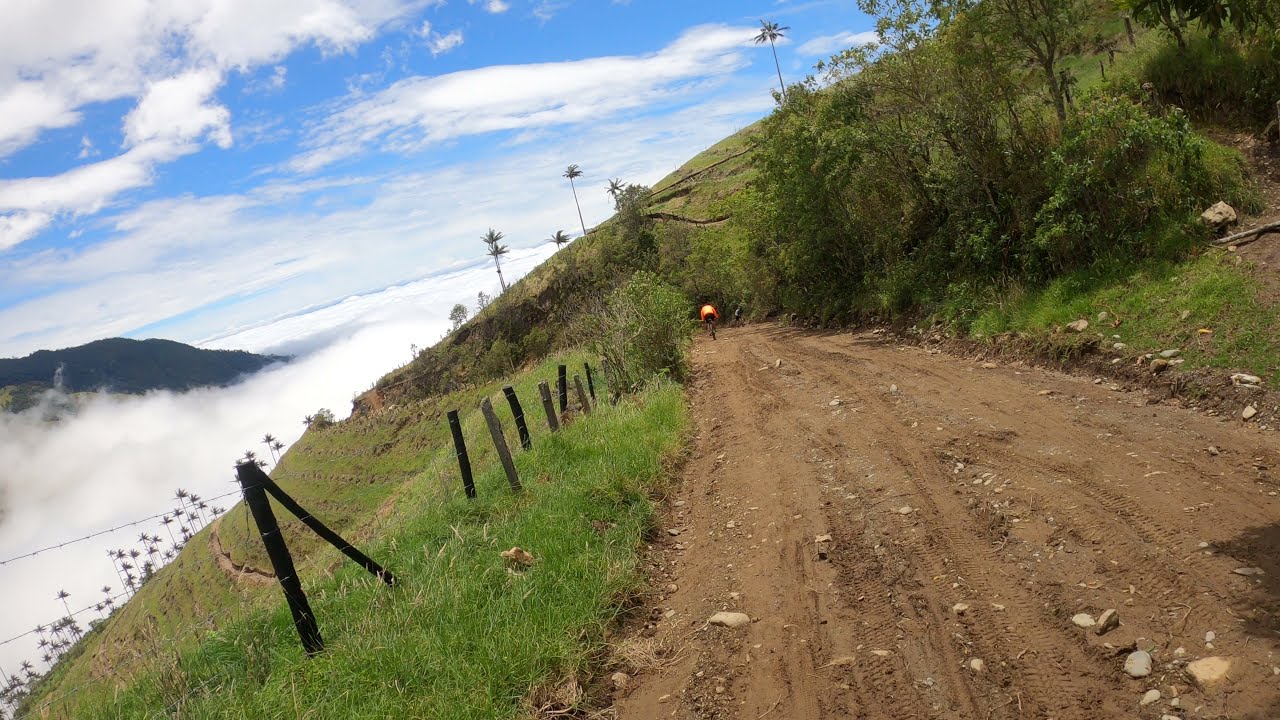In this detailed photograph set at a high elevation during the daytime, we observe a rugged dirt road cutting through the landscape, speckled with rocks and stones. The road winds and angles to the left, eventually disappearing into the hill's slope. Dominating the foreground is a bicyclist dressed in an orange long-sleeved top, facing forward and seemingly ready to navigate the sharp turn. To the left, a dilapidated wooden fence with barbed wire stretches across the slope, its posts emerging sporadically from the bright green grass. On the right, the landscape rises steeply, adorned with scrubby bushes, tall grass, and various trees. Beyond the immediate terrain, we see an expansive mountain peeking through a layer of clouds, emphasizing the high altitude of the scene. The sky above is a vibrant blue, punctuated by fluffy white clouds that underscore the majestic elevation of this serene yet rugged locale.